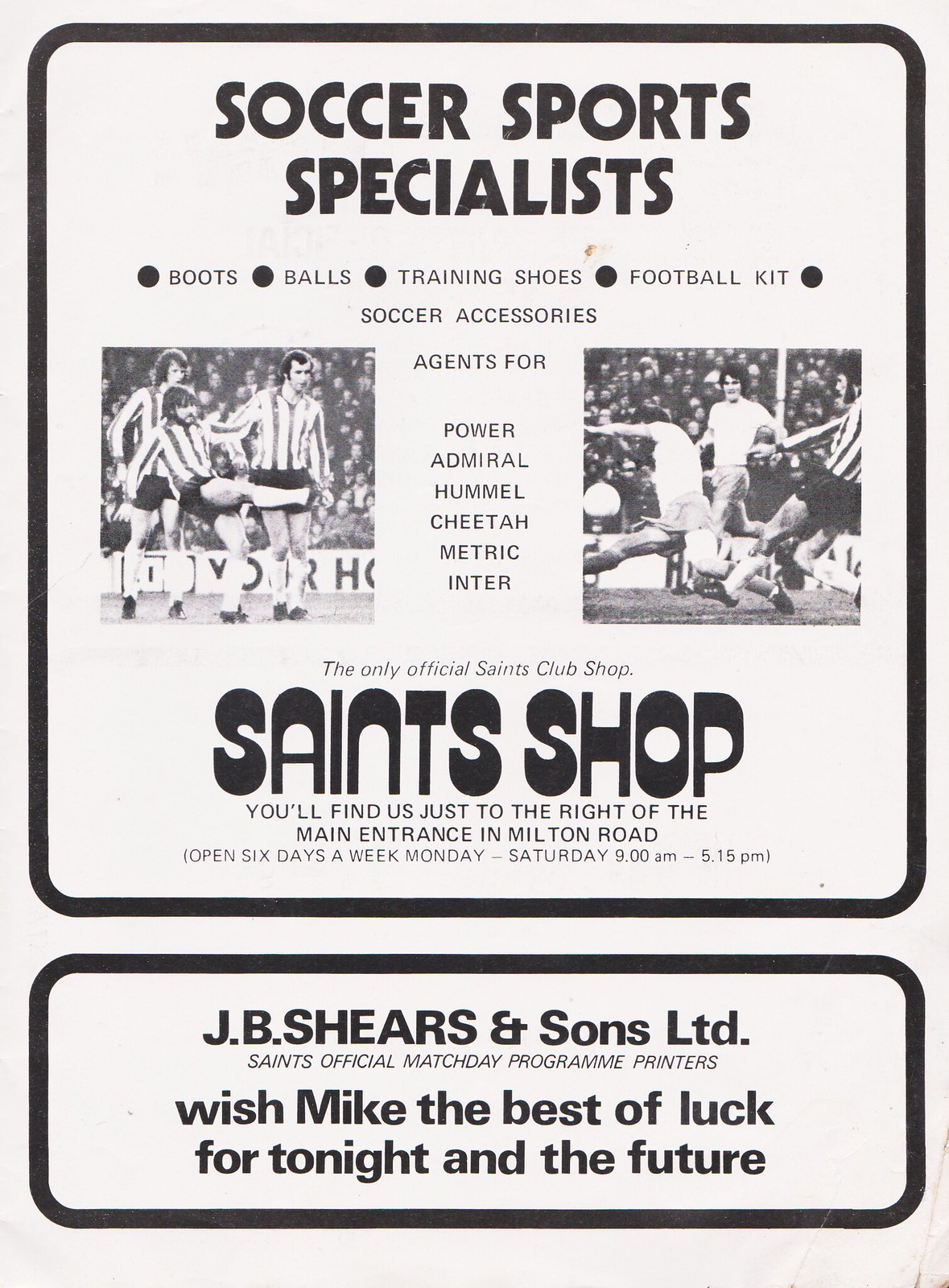This image appears to be a page from an old black-and-white soccer magazine, likely from the 1960s or 1970s. The page is dominated by two text boxes. The larger text box at the top prominently features the title "Soccer Sports Specialists" and lists various soccer-related items such as boots, balls, training shoes, football kits, and soccer accessories. The text also mentions they are agents for multiple brands including Power, Admiral, Hummel, Cheetah, and Metric. Additionally, it highlights that this is "The Only Official Saints Club Shop" and provides location details, stating it's just to the right of the main entrance on Milton Road, and operational hours from Monday to Saturday, 9 a.m. to 5:15 p.m. Accompanying the text are two black-and-white photographs of soccer players in action, placed on either side of the text. 

The bottom text box, which spans the width of the page but is much shorter, states "JB Shears and Sons Limited," identified as the "Saints Official Match Day Program Printers." This text extends well-wishes to a person named Mike for his future, with the phrase, "Wish Mike the Best of Luck for Tonight and the Future." The overall aesthetic is distinctly nostalgic, with a clear vintage quality that emphasizes its era.